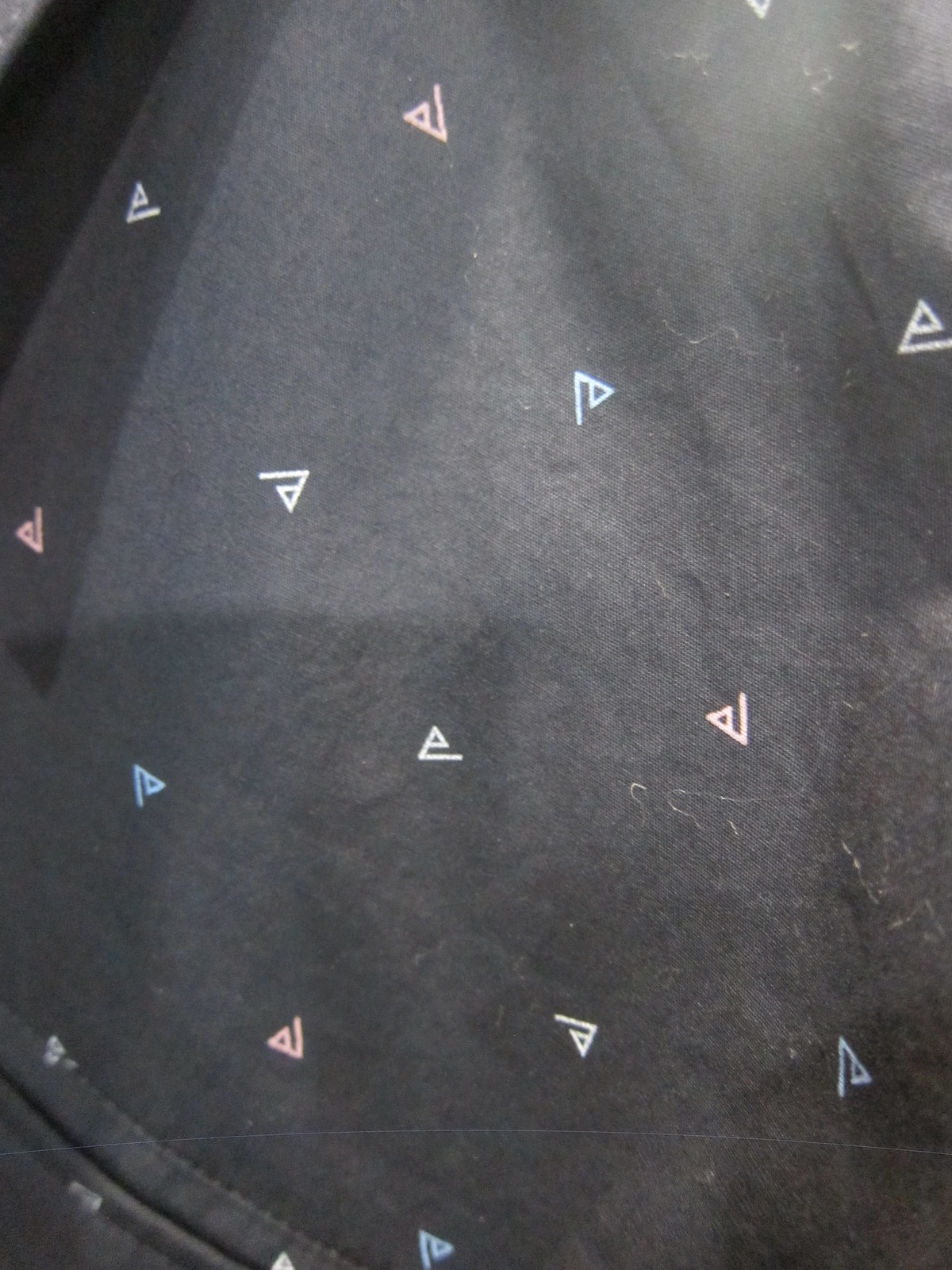This close-up image showcases a black fabric, possibly a shirt, couch, blanket, or article of clothing, adorned with a consistent pattern of small, multicolored triangular shapes. The triangles are approximately a quarter inch in height and length and appear in various shades, including orange, pink, yellow, light blue, dark blue, and white. Each triangle features a unique design, where some look like incomplete triangles with smaller triangles inside them. The fabric itself appears worn and slightly faded, suggesting it has been washed several times. Additionally, a seam, possibly a zipper seam, is visible at the bottom of the image, further indicating it might be a piece of clothing.